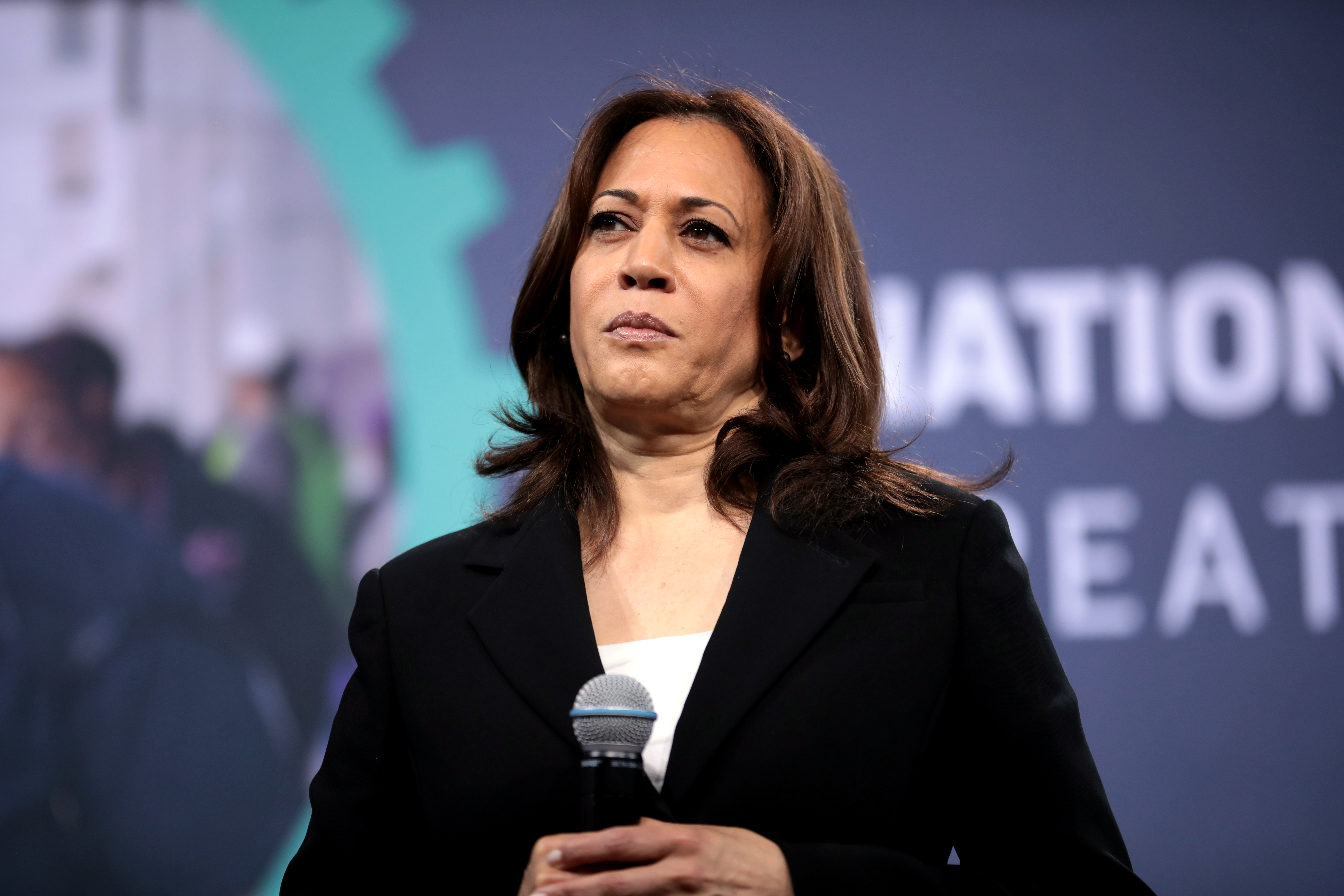In this image, Kamala Harris stands at the center of attention, dressed in a black blazer over a white shirt. Her long, shoulder-length brown hair frames her serious expression as she gazes slightly upwards and to the left. She holds a microphone with both hands, the microphone's black base transitioning to a silver top highlighted by a blue band.

The backdrop is a dark blue panel adorned with large, partially obscured white text, displaying "A-T-I-O-N" and "E-A-T". The left side of the panel features a blurry image that appears to depict a building and people, including a person in a safety vest and white hard hat. A decorative element resembling a curved, teal-blue band separates this image from the rest of the background.

Overall, the image captures Vice President Harris in a moment of poised address, framed by an enigmatic and partially legible backdrop.